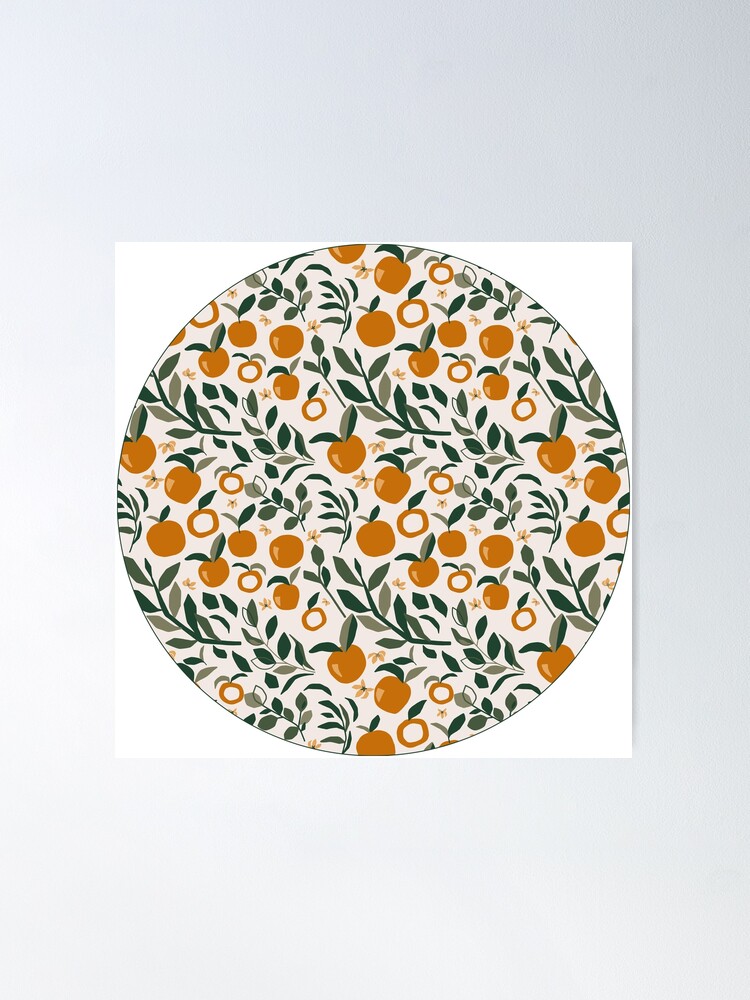The image features a light gray background which occupies the majority of the space. Set against this gray backdrop is a smaller white square. Inside the white square, there is a circular design outlined by a thin black line with a beige background. The circular design is composed of a repetitive pattern of green leaves on stems and small orange fruits. Some of these fruits are solid in different shades of orange, while others are just orange outlines with clear interiors. In addition to the oranges, there are a few small orange flowers interspersed among the leaves and fruits. The pattern covers the entirety of the beige circle, creating a visually appealing abstract artwork that stands out against the simplicity of its surrounding space.